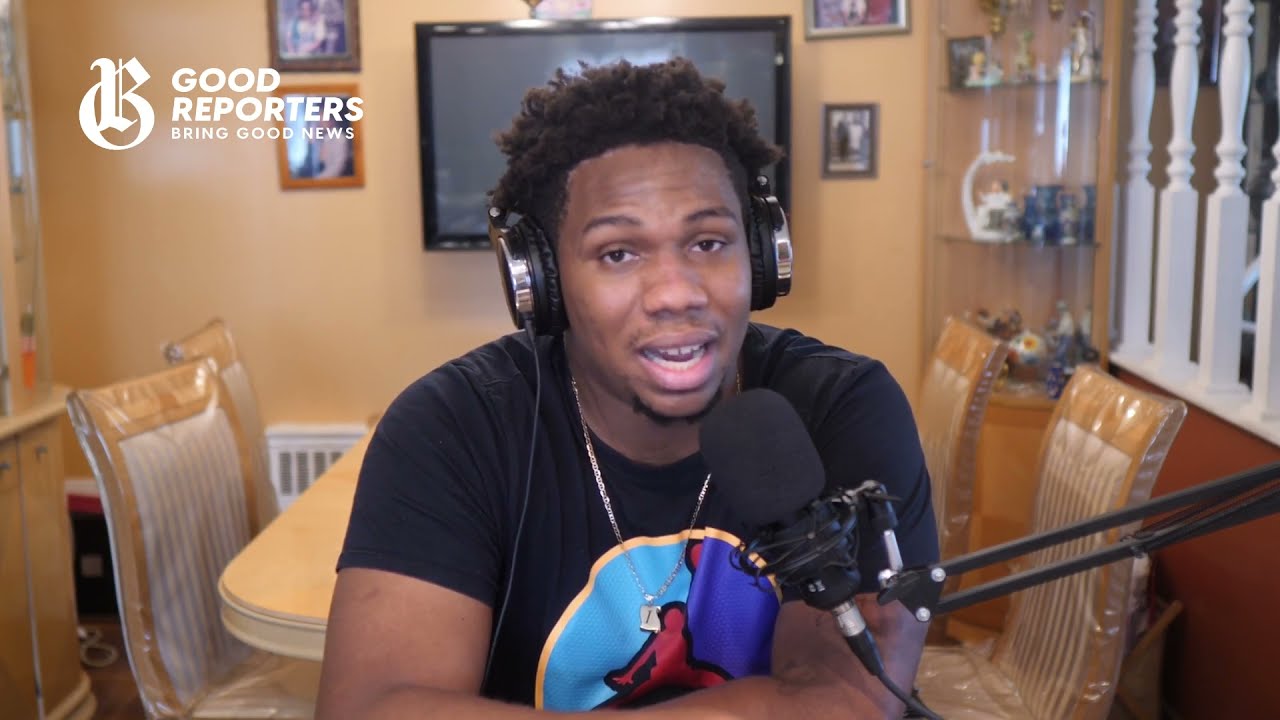The indoor image captures a central view of an African American man speaking into a black microphone with an extending arm, connected by a cord at the bottom. He is wearing large black headphones with chrome accents, a black t-shirt featuring a circular logo resembling the Michael Jordan Jumpman Nike logo, adorned with a red basketball player set against a purple and light blue gradient background, highlighted by a golden border. A silver necklace with a small square ornament rests on his chest. The man’s hair is short but voluminous, and he sports a thin connect beard and mustache (goatee). His mouth is open, mid-sentence.

Behind the man, the dining room setting features a table mostly obscured by his figure, surrounded by four chairs wrapped in plastic and crafted from light wood with cream backs. Mounted on the cream-colored wall directly behind him is a large, black flat-screen TV that’s turned off and almost entirely blocked by his head. The wall showcases framed pictures of a couple, flanking the TV. On the right, a china cabinet filled with various knickknacks occupies a corner of the room. Vertically placed white railings suggest the presence of a nearby staircase. The upper left of the image contains a logo that reads "Good Reporters Bring Good News" in white font, along with a cursive "R" transitioning into a zero.